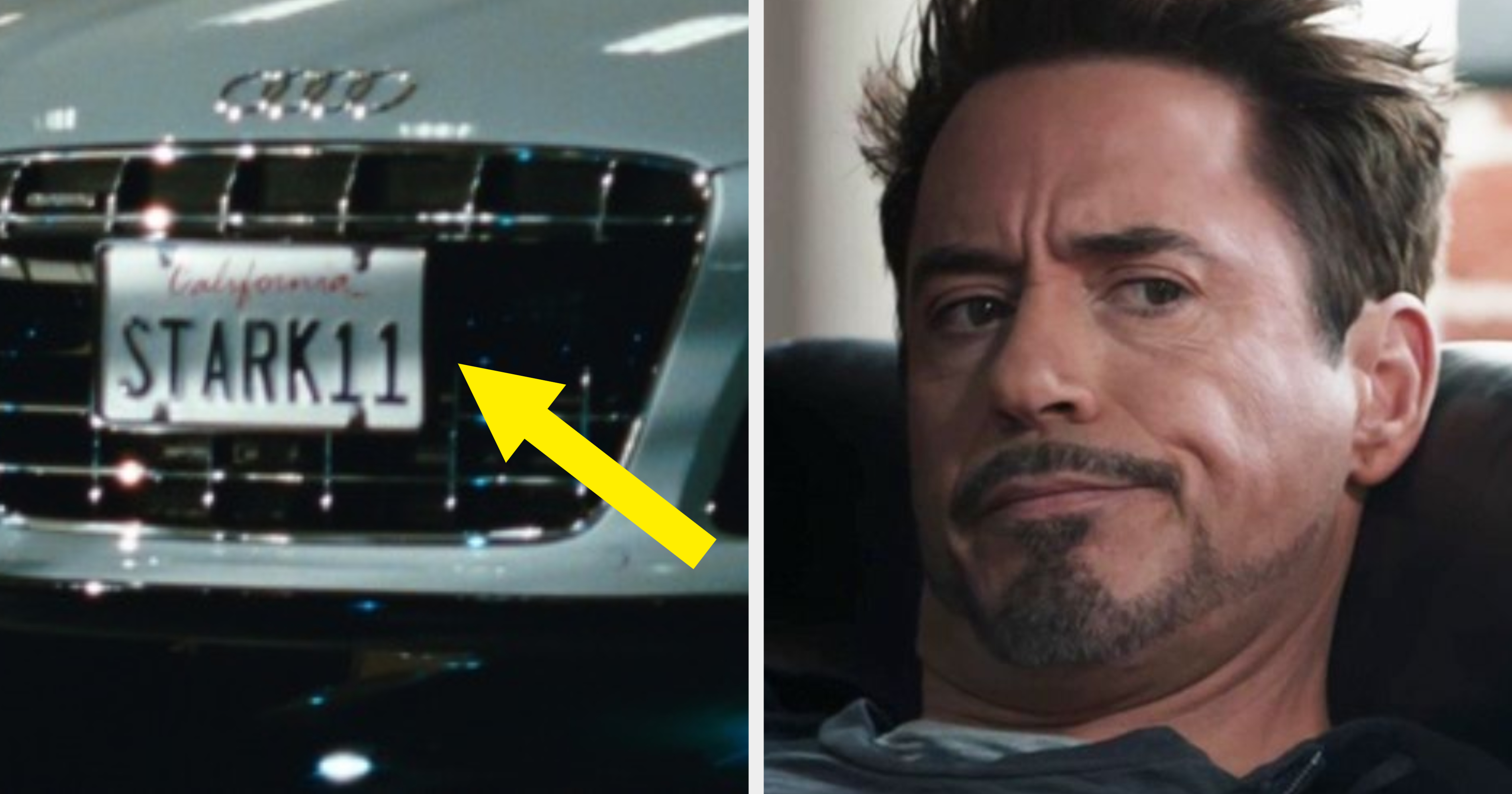The image is divided into two panels. On the left, there is a close-up of the front portion of a white Audi car, showcasing its silver grill and the iconic four-ring Audi logo. Prominently displayed is a white California license plate with "California" inscribed in red cursive at the top and "STARK 11" printed in bold blue capital letters at the bottom. A yellow arrow is superimposed over the image, pointing downward diagonally towards the license plate. On the right side, we see Tony Stark, portrayed by Robert Downey Jr., displaying a disgruntled expression with his brows furrowed and one side of his mouth raised in a smirk. He has brown hair, brown eyes, and a stylized goatee. Stark appears to be sitting down, possibly on a couch or chair, wearing attire that is dark-colored and somewhat indeterminate due to the angle and lighting. He is looking off-screen, seemingly skeptical or displeased with the information he is receiving.